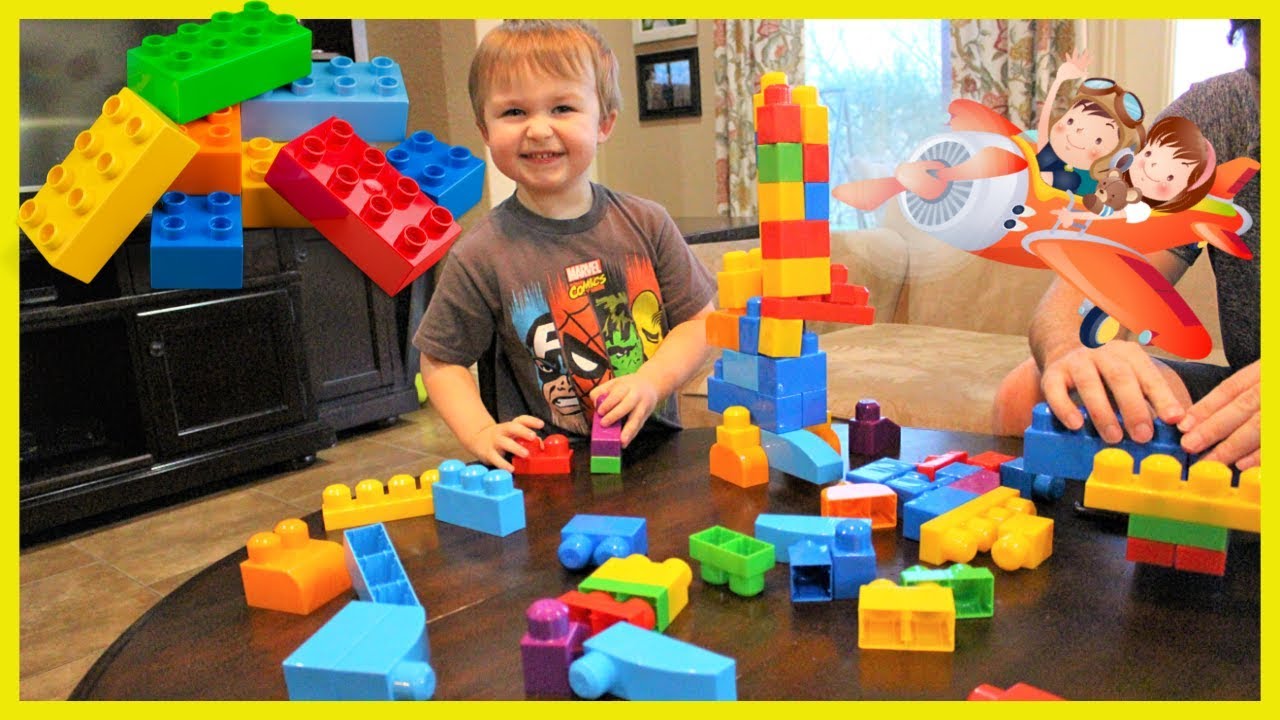This photograph captures a cheerful little boy, approximately 4 or 5 years old, with short blonde hair, smiling at the camera. He is wearing a gray t-shirt that features the Marvel Comics logo along with characters like Captain America, Spider-Man, The Hulk, and Iron Man. The boy is immersed in building a tower or robot using oversized, brightly colored Lego-like blocks on a polished, circular wooden table, which also has a small crack. The blocks are scattered across the dark wood surface and display a range of colors such as blue, green, yellow, red, and purple. To his right, an adult male—likely his father—is also engaged in the activity, constructing something with the blue blocks. The living room backdrop includes a tan couch, a black entertainment center with a television on the left, and two white curtains adorned with vine patterns. Additionally, in the upper left corner of the image is a stack of Legos, while in the upper right, there is a small cartoon airplane with an orange and white color scheme, depicting a boy and a girl inside. The floor is paved with brown stone tiles.